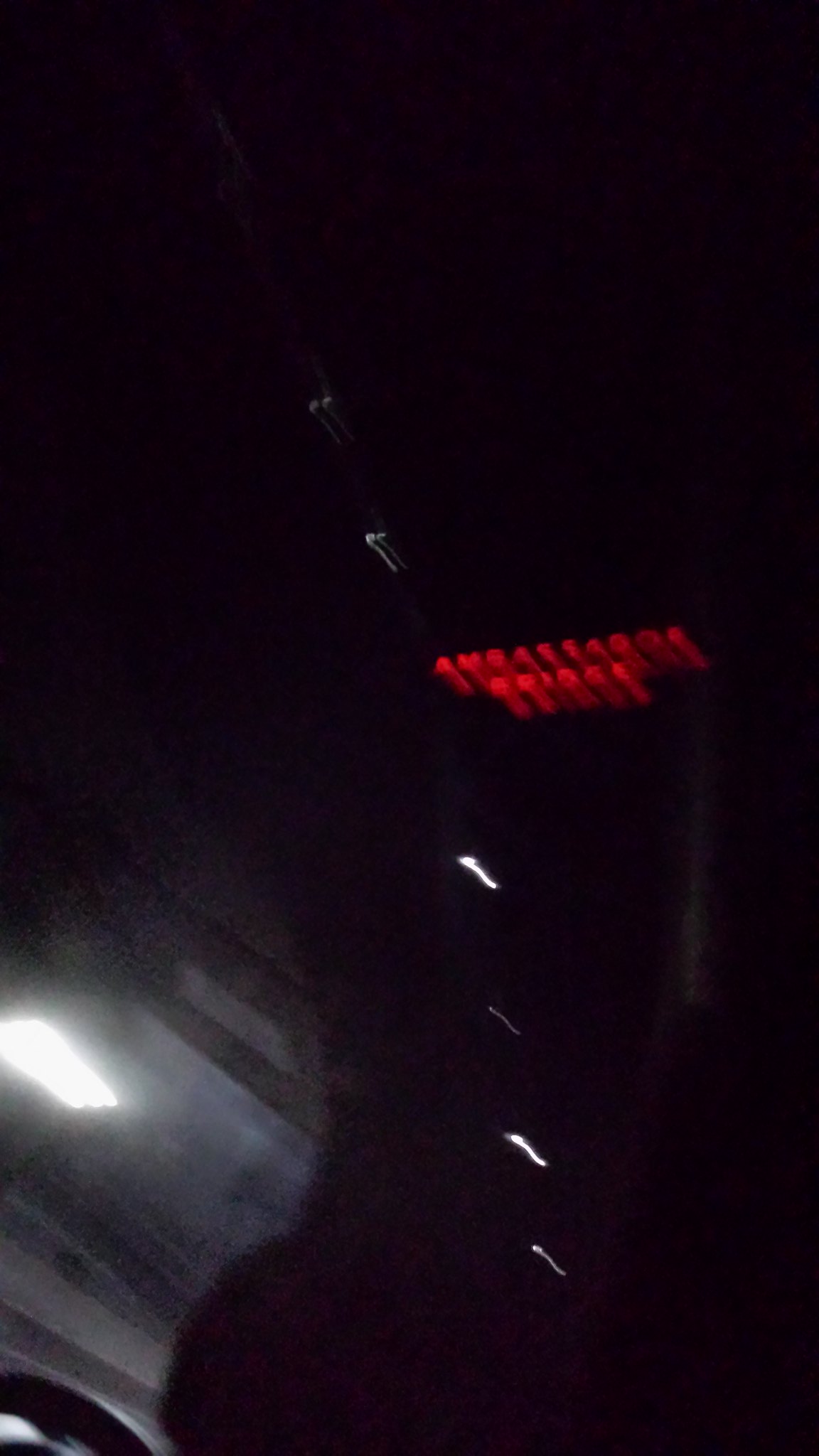A dimly captured photograph presumably taken at night, featuring a prominent sign illuminated by red neon lights spelling "Ambassador Bridge". The neon lights reflect a hazy, red glow, creating an abstract and blurry visual. Below the sign, there are several small, illuminated lines whose details are obscured by the poor image quality. To the bottom left of the image, there's a brilliant white light, accompanied by an indiscernible glowing object, adding to the mystique of the nighttime scene.